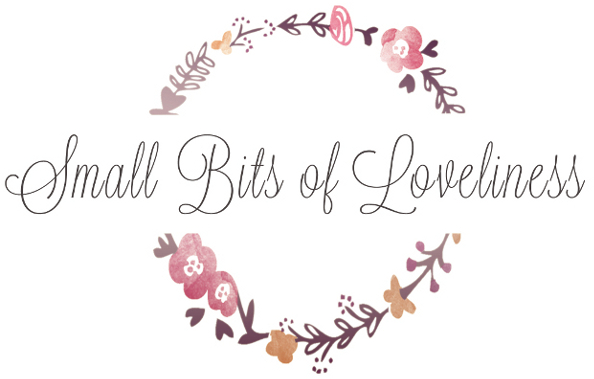The image features a logo set against a solid white background. Central to the design is a circular floral wreath that is beautifully crafted with an assortment of elements such as flowers, petals, leaves, and hearts. This circular pattern is interrupted at the middle by a piece of text which reads "small bits of loveliness" in a narrow, ornate cursive font. The wreath includes colors such as purple, pink, brown, and black, with the top arc of the wreath curving from the lower left to the upper right and adorned with flower petals and various shaped leaves. Similarly, the bottom arc curves in the opposite direction and features larger flower petals and bigger brown leaves. The floral elements also contain heart shapes and are composed in a way that suggests stylization, possibly with dots adding to their texture. The overall appearance is that of a meticulously detailed design, both in its floral motifs and its elegantly written text.